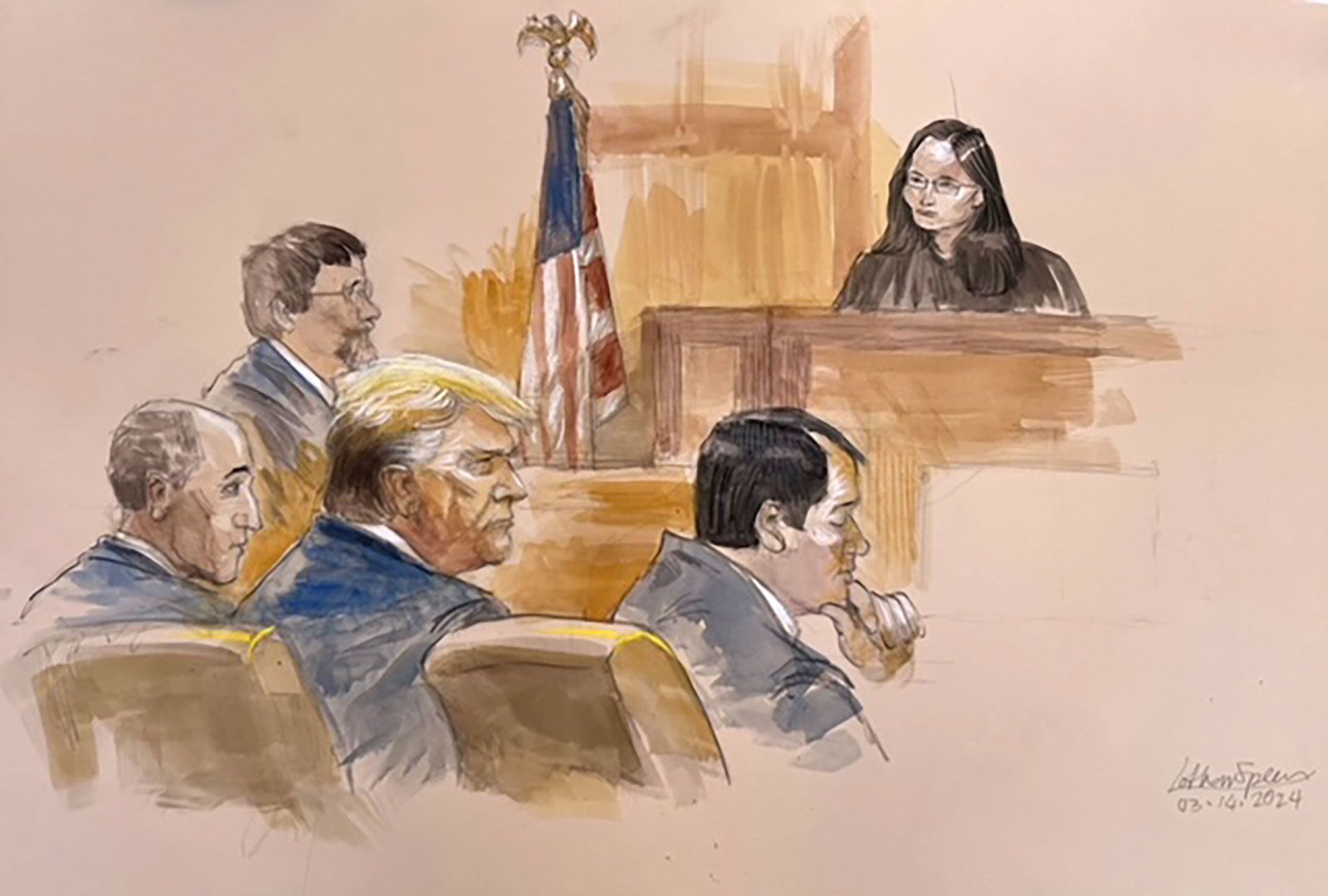This detailed courtroom drawing, in a watercolor style, captures a tense scene featuring Donald Trump scowling in profile as he sits between two men, presumably his lawyers, who are all dressed in blue suits. Trump's prominent reddish blonde hair is notable against his blue jacket. The man to his right, with dark hair and a gray jacket, leans forward, resting his chin on his left hand. On Trump's left side is a balding man, also in a blue suit. The background reveals a man with brown hair and glasses, positioned left to right in profile, suggesting he might be an observer or witness. Above and left of Trump, presiding over the courtroom, is a female judge with long, dark hair, small glasses, and potentially Asian features, wearing a traditional black robe. An American flag with an eagle on top of the pole stands to the right of the judge's elevated wooden desk. The scene is completed by a signature at the bottom right corner, possibly reading "Helen Spears 3-16-2024," written in cursive and difficult to discern. The chairs and desk in the courtroom are rendered in brown, providing a cohesive background for the figures.